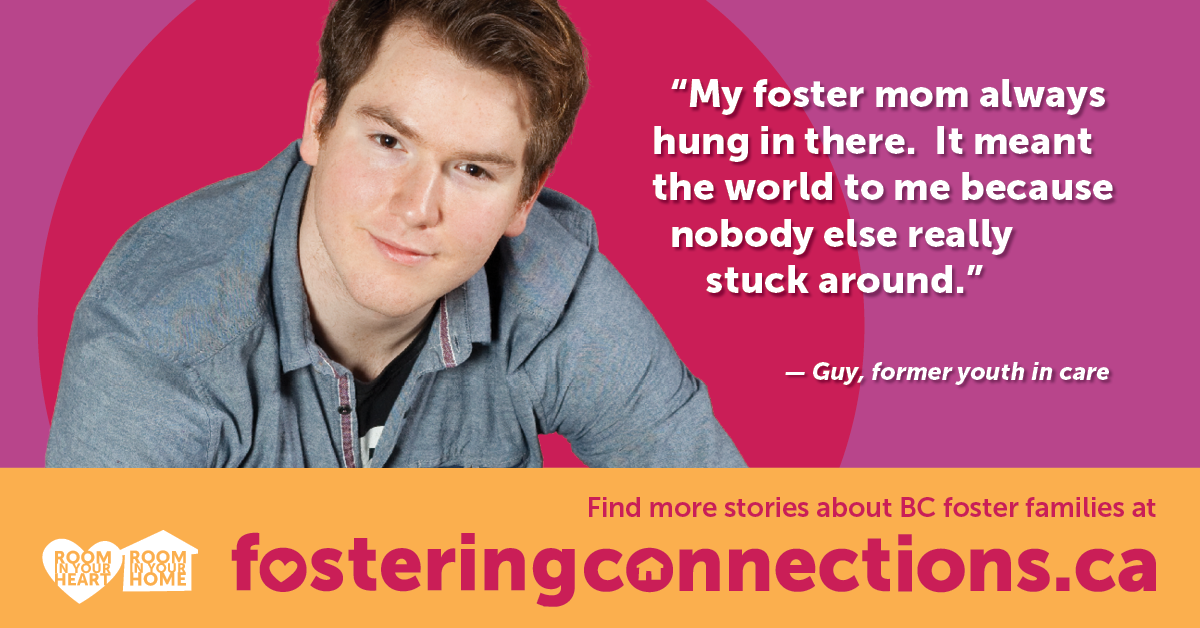The poster for Fostering Connections features a young adult white male prominently on the left-hand side against a purple background with a red circle behind him. Positioned to the right of the young man is a heartfelt quote in bold white text: "My foster mom always hung in there. It meant the world to me because nobody else really stuck around," attributed to Guy, a former youth in care. At the bottom of the poster, there is a horizontal rectangle with an orange background bearing red text that reads "FosteringConnections.ca" and "Find more stories about BC foster families at FosteringConnections.ca". On the bottom left of the poster, there is a white heart inside a white house accompanied by orange text that says "Room in your heart, room in your home."